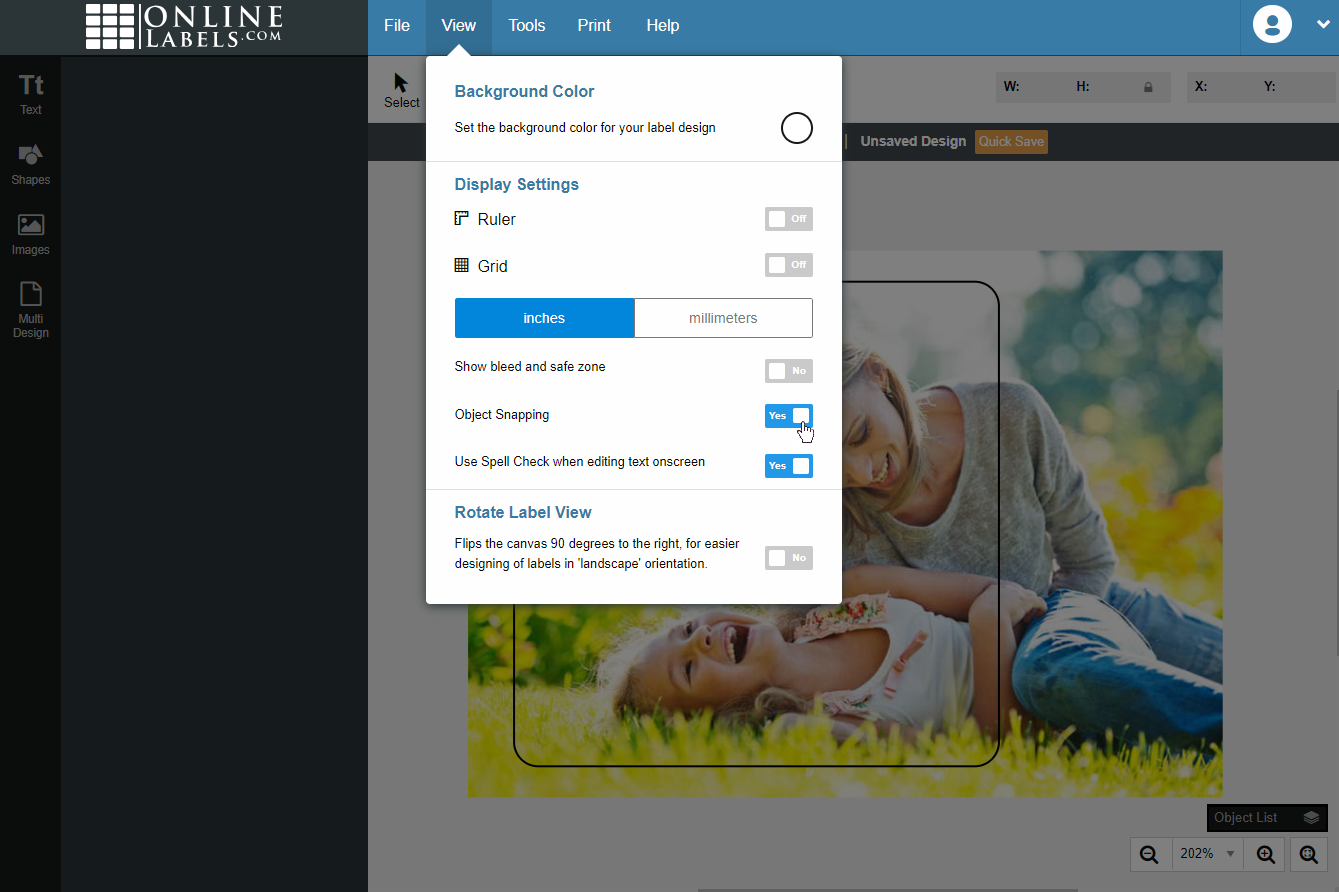This image is a detailed screenshot from a web page belonging to onlinelabels.com. In the top-left corner, there is a logo that identifies the website. Adjacent to the logo, a blue navigation bar features options such as File, View, Tools, Print, and Help. The View tab is currently selected, revealing choices for customizing the display settings.

The chosen background color for the display is white. Other available settings include metrics for Display Preferences, with 'ruler' and 'grid' configured to display measurements in inches. The options to 'Show Bleed' and 'Safe Zone' are turned off, while 'Object Snapping' and 'Use Spell Check When Editing Text On-Screen' are enabled. Additionally, the feature to 'Rotate Canvas 90 Degrees to the Right' for easier landscape label design is disabled.

Beneath this interface, on the left side of the webpage, a black sidebar extends vertically down the screen. The larger central section of the screen showcases the main design area, which features a photograph. In the image, a woman and a young girl, both dressed in jeans, are lying on grass in a meadow. The young girl is wearing a white shirt adorned with pink flowers, while the woman dons a gray long-sleeve T-shirt. The serene background includes greenery and out-of-focus trees, adding a tranquil natural setting to the scene.